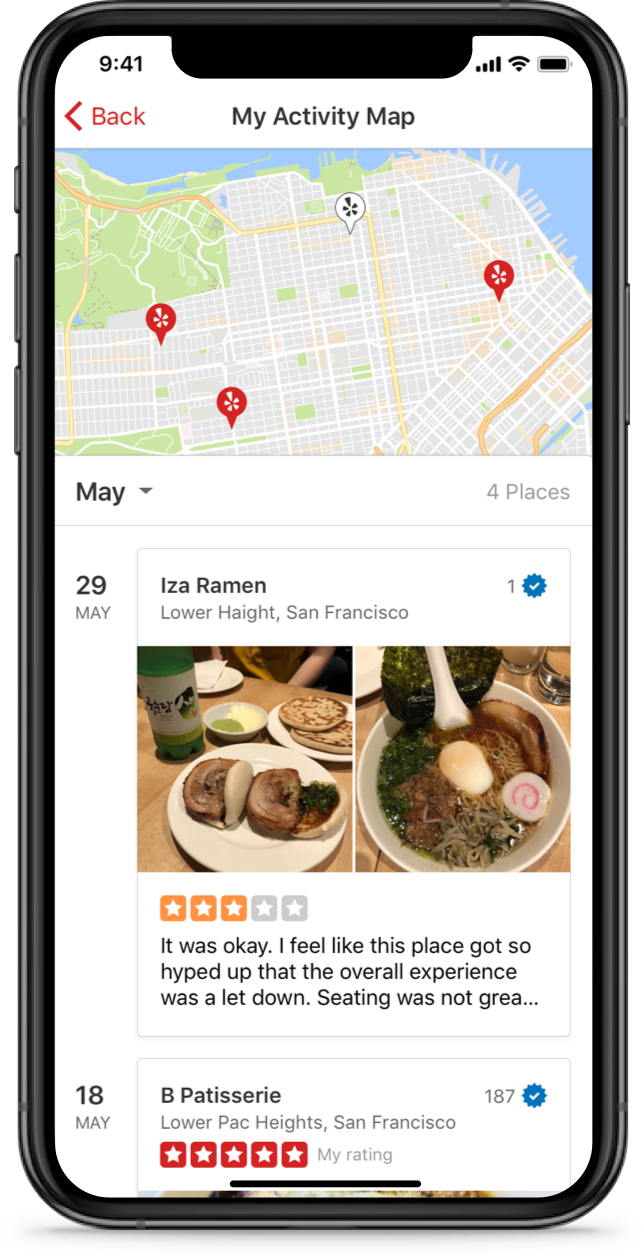The image displays a smartphone screenshot with a black border. At the top, the status bar shows the time "9:41" alongside four full signal bars, a full Wi-Fi signal icon, and a fully charged battery icon. Beneath the status bar, a red arrow symbol (<) labeled "Back" is followed by the title "My Activity Map" in black text.

The main content area features a Google Maps screenshot marked with four location pins: one white and three red, scattered over an unspecified location. Below the map, the interface presents a dropdown menu labeled "May" showing "4 places" and a specific date, "29 May."

Further down, detailed information about a visit to a place called "Eyes of Ramen" located in Lower Heights, San Francisco, is provided. This includes two photographs of food served on plates atop a table, accompanied by a rating of "3 out of 5 stars." The user review states: "I said it was okay, I feel like this place got so hyped up that the overall experience went a lot down. Seating was not great."